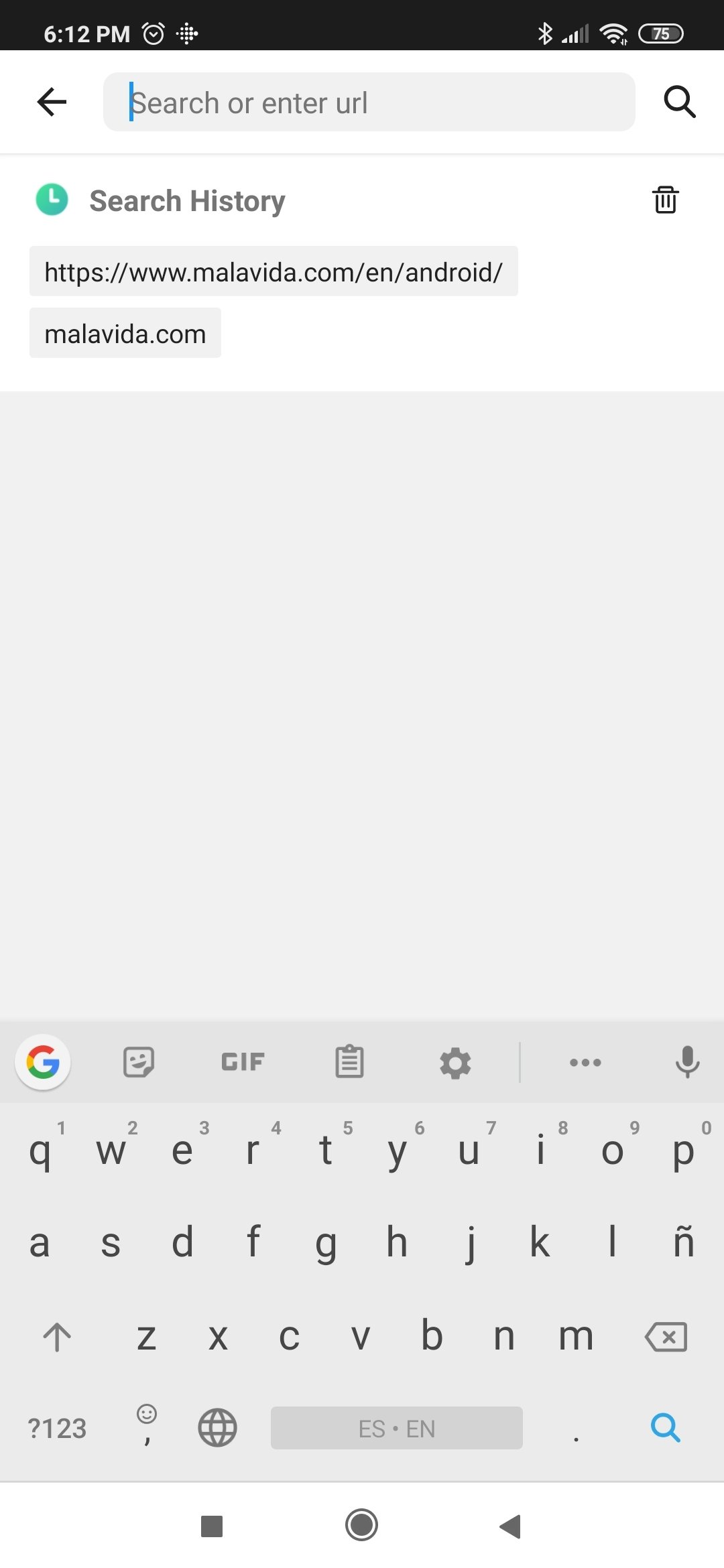This detailed caption precisely describes the elements visible in a screenshot of a cell phone's browser search interface:

---
A screenshot of a cell phone displays a web browser interface. At the top of the screen is a search bar with a back arrow icon on the left. The search bar contains a blinking blue cursor, indicating it is active. On the right side of the search bar is a magnifying glass icon, signifying the search function. Below the search bar, the screen shows search history with a clock icon on the left followed by the text "Search history." Underneath, there is a URL displayed: "https://www.malavita.com/EN/Android," with the website name “malavita.com” listed below it. A gray empty square is visible beneath the URL section. At the bottom of the screen, the cell phone's on-screen keyboard is displayed, featuring the standard keys along with a Google button and a GIF icon positioned just above the keyboard.
---

This caption provides a thorough and organized overview of all the details visible in the photo.